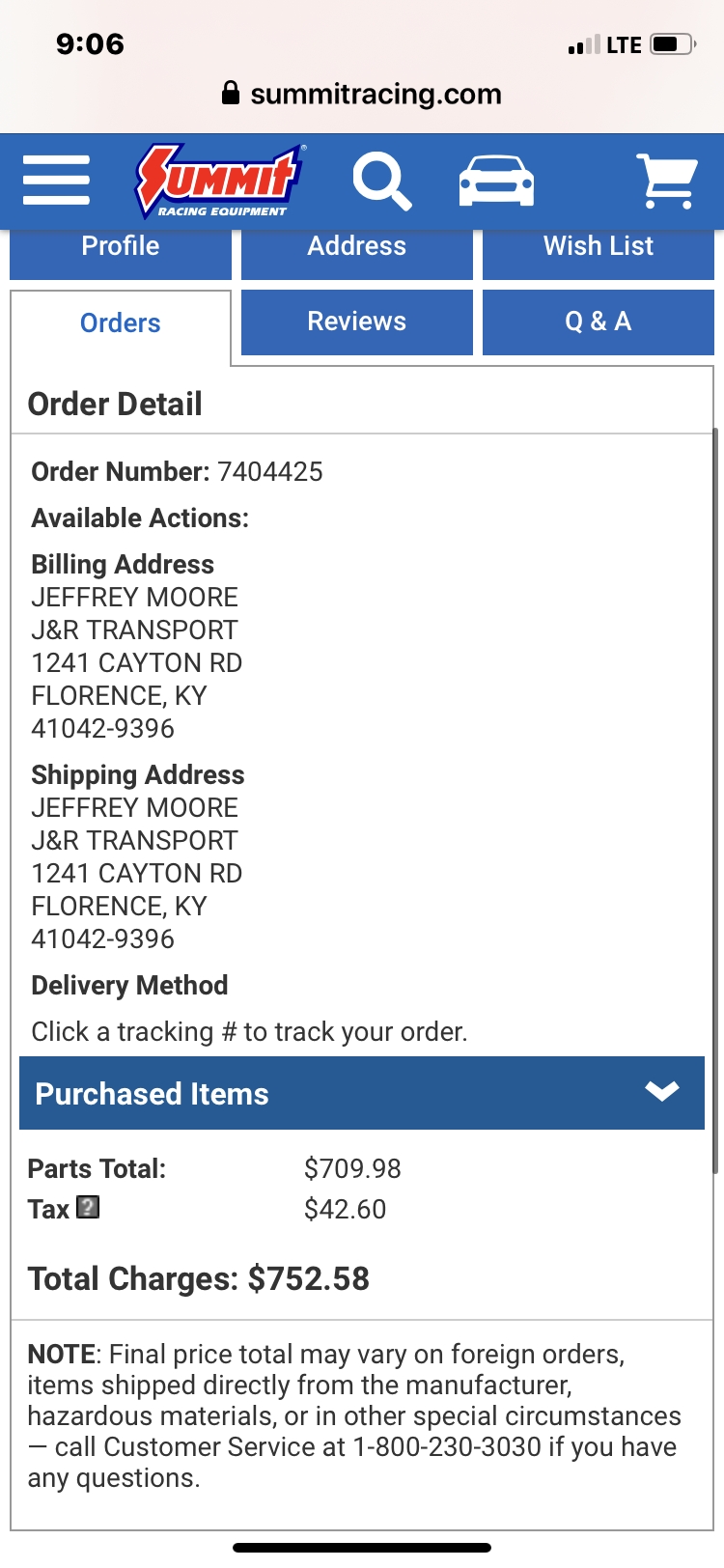**Screenshot Description: Summit Racing Mobile Interface**

A screenshot taken from a mobile phone displays the Summit Racing website at 9:06 AM. The phone shows 2 out of 4 signal bars and about 75% battery life remaining. 

The image features the Summit Racing website with a distinctive blue header at the top. "Summit" is prominently displayed in red letters. To the right of the logo are icons for search (magnifying glass), categories (car icon), and shopping cart.

Below the header, several options are listed as buttons: "Profile," "Address," "Wishlist," "Orders," "Reviews," and "Q&A." 

Under the "Orders" section, the screen details an order history: 

- **Order Detail:**
  - **Order Number**: 7404425
  - **Available Actions**

- **Billing Address:**
  - Jeffrey Moore, J&R Transport
  - 1241 Caton Road, Florence, KY 41042-9396

- **Shipping Address:**
  - Jeffrey Moore, J&R Transport
  - 1241 Caton Road, Florence, KY 41042-9396

- **Delivery Method:**
  - Click a Tracking Number to track your order

- **Purchase Items:**
  - Parts Total: $709.98